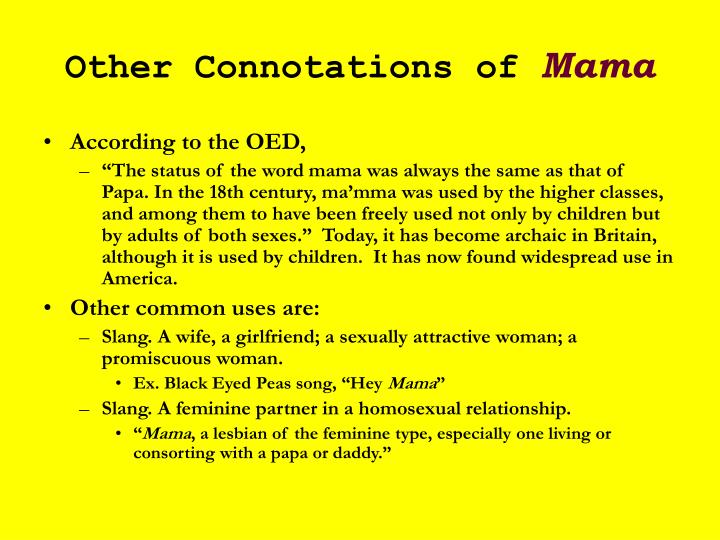The image depicts a yellow slide from a larger presentation, focusing on the word "mama" and its various connotations. The slide is titled "Other Connotations of Mama," with "mama" highlighted in maroon ink, and the rest of the title in black ink. The content is organized into two main bullet points.

The first bullet point, beginning with "According to OED," explains the historical status of the word "mama." It details that in the 18th century, "mama" held the same status as "papa," being used by the higher classes and not only by children but also adults of both sexes. Today, the term has become archaic in Britain but remains in widespread use among children in America.

The second bullet point lists other common and slang uses of the word "mama." These include references to a wife, a girlfriend, a sexually attractive woman, or a promiscuous woman—citing examples like the Black Eyed Peas song "Hey Mama." Additionally, it mentions "mama" as slang for a feminine partner in a homosexual relationship, specifically a lesbian of the feminine type, who may live or consort with a "papa" or "daddy."

Overall, the detailed slide appears to be part of a linguistics presentation or conference, emphasizing the diverse meanings and social implications of the word "mama."